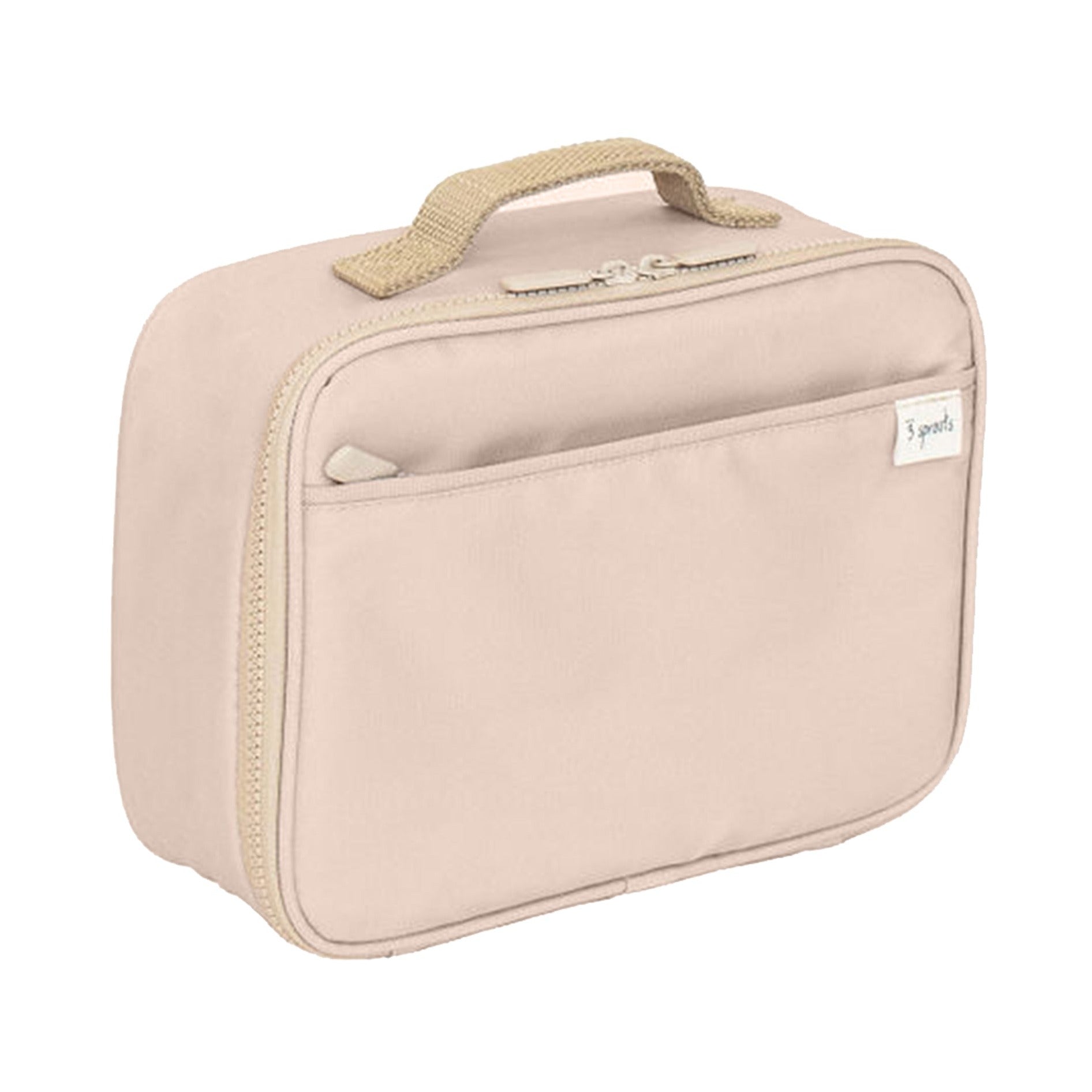A small, rectangular-shaped bag with curved corners and a very light pink, almost pastel, color is featured in this image. The bag, which could potentially be a purse, camera sack, makeup bag, or toiletry bag, is positioned with its front side slightly facing right, revealing multiple details. 

The top of the bag has a double zipper system that allows it to open towards the center, with zippers that appear to be beige in color. On the front side, there's an additional pocket with a visible zipper tag. Another notable feature is a white label on the right side with the text "Three Sprouts" and a logo beside it, though the words are somewhat hard to read.

The bag also has a handle, described variably as a wrist strap, hand strap, or braided handle, in a light brown or beige color. This handle is situated on the top of the bag. Overall, the small bag is placed against a white surface with a white background, making the soft pink color stand out prominently.